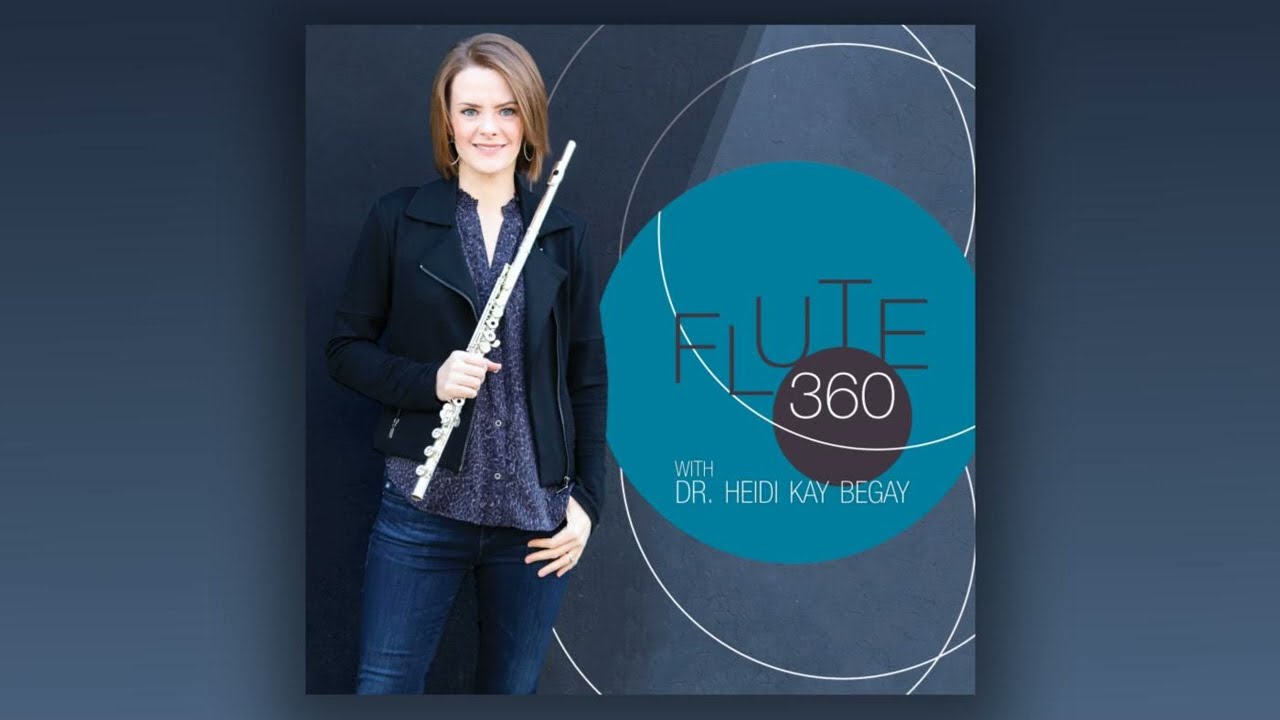The image features a Caucasian woman standing slightly to the left, holding a silver flute diagonally across her body with her left hand, the instrument extending over her right shoulder and down to her left hip. She has light brown hair, parted on the left side, and cut just below her jawline. She is smiling, showing her red cheeks and blue eyes. She is dressed in a black leather jacket with a thick collar and an open zipper, underneath which she wears a blue button-up shirt adorned with floral patterns, forming a V-neck at the top. She also has blue jeans on and accessorizes her look with large silver hoop earrings. The woman's right thumb is casually tucked into her jeans pocket. To her right is a teal-colored circle with the word "FLUTE" in black letters, inside of which is a smaller black circle detailing "360" in white font. Below this smaller circle, white text reads "With Dr. Heidi K. Begay." The backdrop features a banner promoting the event "Flute 360 with Dr. Heidi K. Begay," accentuated with white circular lines throughout the background.